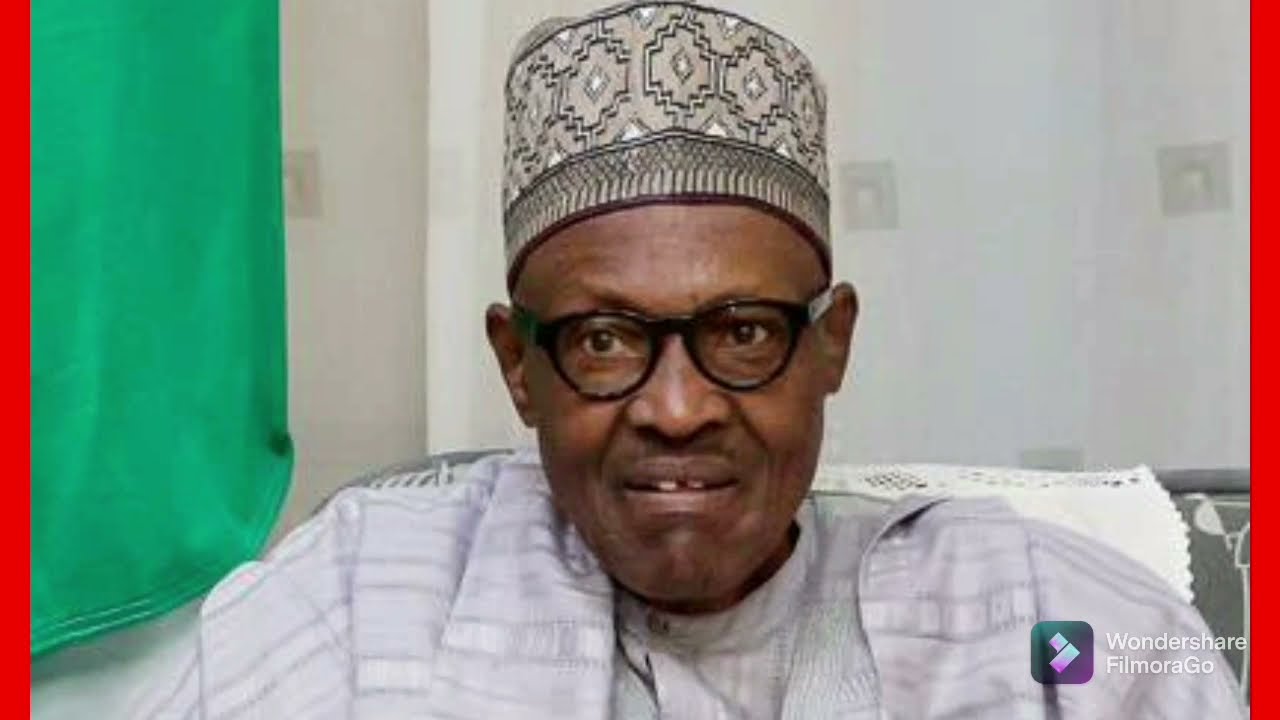The image portrays an older African gentleman with a shaved head sporting a traditional, intricately designed gray African hat adorned with white or silvery geometric patterns and possible beading. His expression is serious, with slightly open lips revealing a gap between his front teeth. He wears black, round glasses framing his brown eyes. The man is clad in a gray outfit featuring subtle horizontal stripes and possibly layered with a white or light lavender shawl or robe. He's seated on something gray covered with a white doily. The background consists of a white wall with gray squares and a green curtain with a red trim on the left. In the lower right corner of the image, there is a watermark reading "Wondershare Filmora Go" accompanied by a small square logo divided into a green upper half and a purple lower half with an interlaid L-shaped white design.